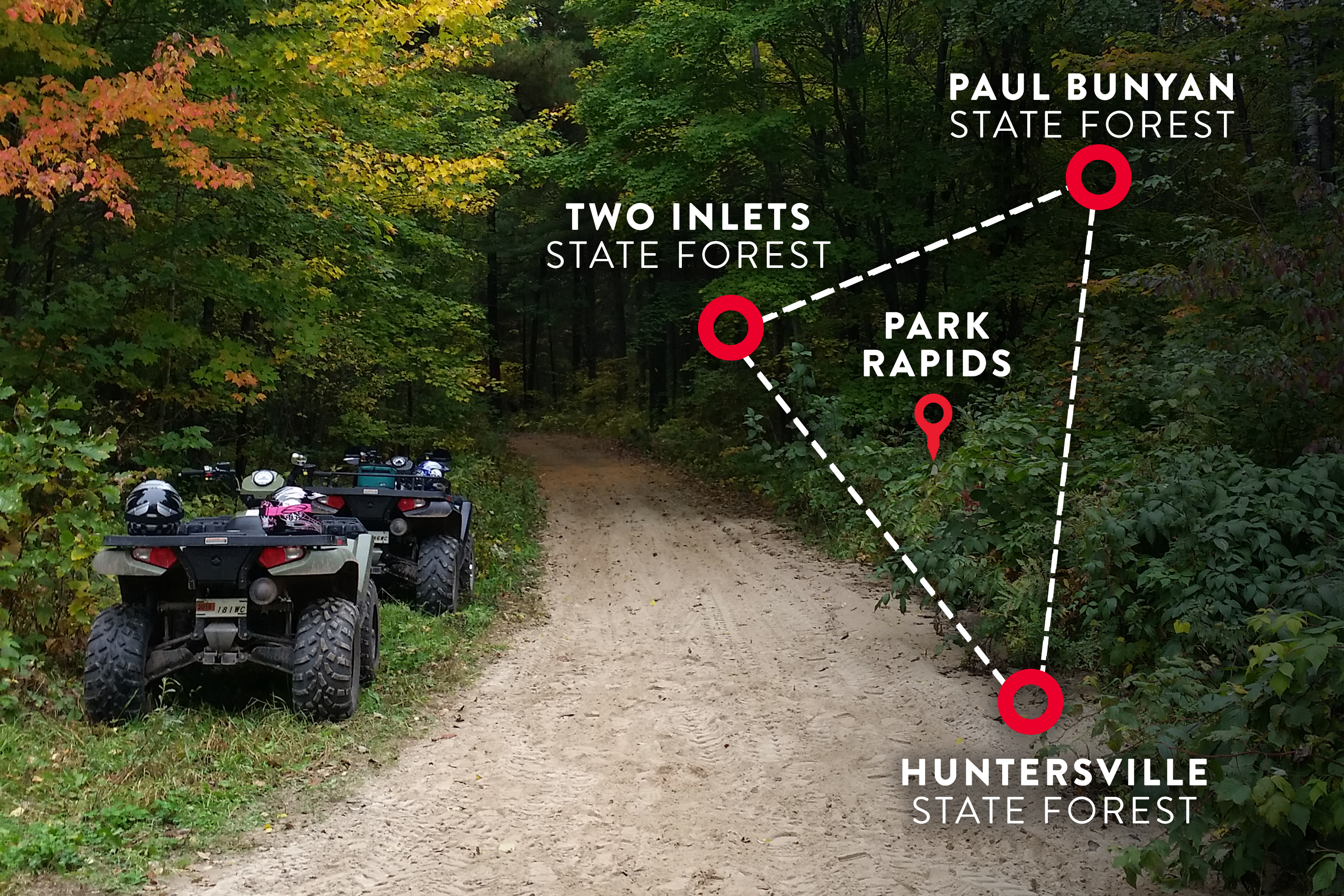The image showcases a forest trail scene featuring two all-terrain vehicles (ATVs) parked one behind the other on a dirt and sand path. The ATV in the back is light green with a black and white helmet, while the one in front is darker green with no helmet. Both vehicles are nestled on a grassy area next to the trail, surrounded by trees, indicating the start of a forest. Centrally, a single-lane road stretches straight ahead. Overlaid on the right side of the image is a detailed map outlining the forest regions, marked by a triangular graphic with dashed white lines and three red circles. Each vertex of the triangle denotes a different state forest: Two Inlets State Forest to the left, Paul Bunyan State Forest at the top right, and Huntersville State Forest at the bottom. A "You Are Here" marker points to Park Rapids within this triangular zone. The colors captured in the image range from forest greens, oranges, and yellows to lighter dirt tones, blacks, whites, grays, blue-green hues, and pink.